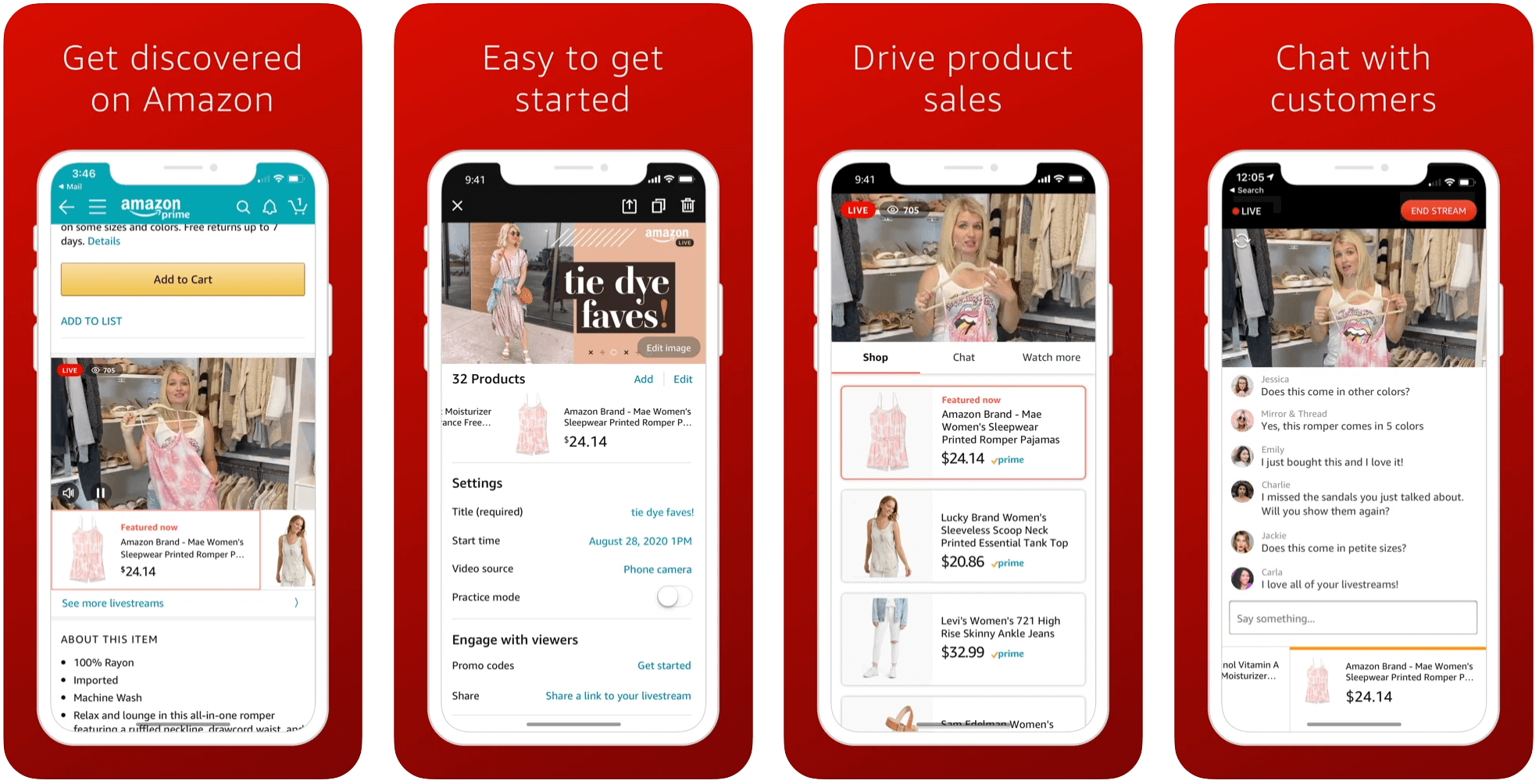This composite image features four screenshots from Amazon, each capturing a different aspect of the online shopping experience for women's apparel. 

The first screenshot highlights the product page for the "Maywoman Sleepwear Printed Romper," priced at $24.14. Key features are listed, including its composition of 100% rayon, its imported origin, and the recommendation for machine washing. The product description suggests it is perfect for relaxing and lounging, featuring a ruffled neckline and a drawcord waist. Options to "Add to Cart" and "Add to List" are prominently shown, along with tags such as "Featured Now" and "Amazon Brand."

The second screenshot displays a selection labeled "Tie-Dye Faves," featuring two different tie-dye patterned products, appealing to the trending fashion interest of customers.

The third screenshot showcases three different items: the "Maywoman Sleepwear," the "Lucky Brand Women's Sleeveless Neck Printed Essential Tank Top," and the "Level's Women 7 to 1 High Rise Skinny Ankle Jeans." These items collectively imply a versatile mix-and-match wardrobe for various occasions.

The fourth screenshot consists of user questions and comments, providing insight and reviews from previous purchasers, aiding potential buyers in making informed decisions about the products.